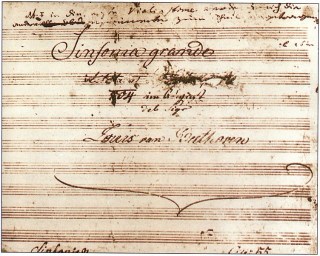The image appears to depict an aged sheet of music, rendered in dark red ink on what resembles a cream-colored, parchment-like background, adding to its antiquated appearance. The sheet is lined like a musical staff but contains no visible musical notes, only text that is neither legible nor in a recognizable language. The calligraphy is ornate, suggesting it might be an invitation to a sophisticated event, possibly a concert, with the words "Symphony Grand" standing out amid the faded and blurred text. Towards the bottom, an elegant, curly-Q design embellishes the page, enhancing its vintage aesthetic. The overall condition, with its dingy white and brownish hues, gives the impression that the piece dates back to the 1800s, captured in a small, detailed photograph.